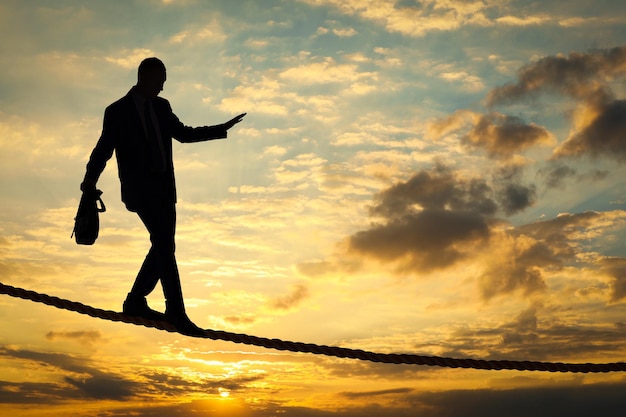The image captures a striking silhouette of a man walking carefully on a slightly downward-sloping tightrope against a breathtaking sunset. The sky transitions from a deep blue at the top, scattered with white fluffy clouds, to a brilliant golden hue near the horizon where the sun is setting. Dark, blackish-gray clouds accentuate the sky's dramatic palette. The man, appearing as a stark black shadow, seems to be wearing a suit, with long sleeves and pants, and possibly pointy shoes. He carries a bag in his outstretched right hand, while his left hand is held slightly behind him, aiding his balance. His cautious steps suggest a sense of focus and determination as he navigates the woven rope, which stretches from left to right, cutting through the radiant backdrop.